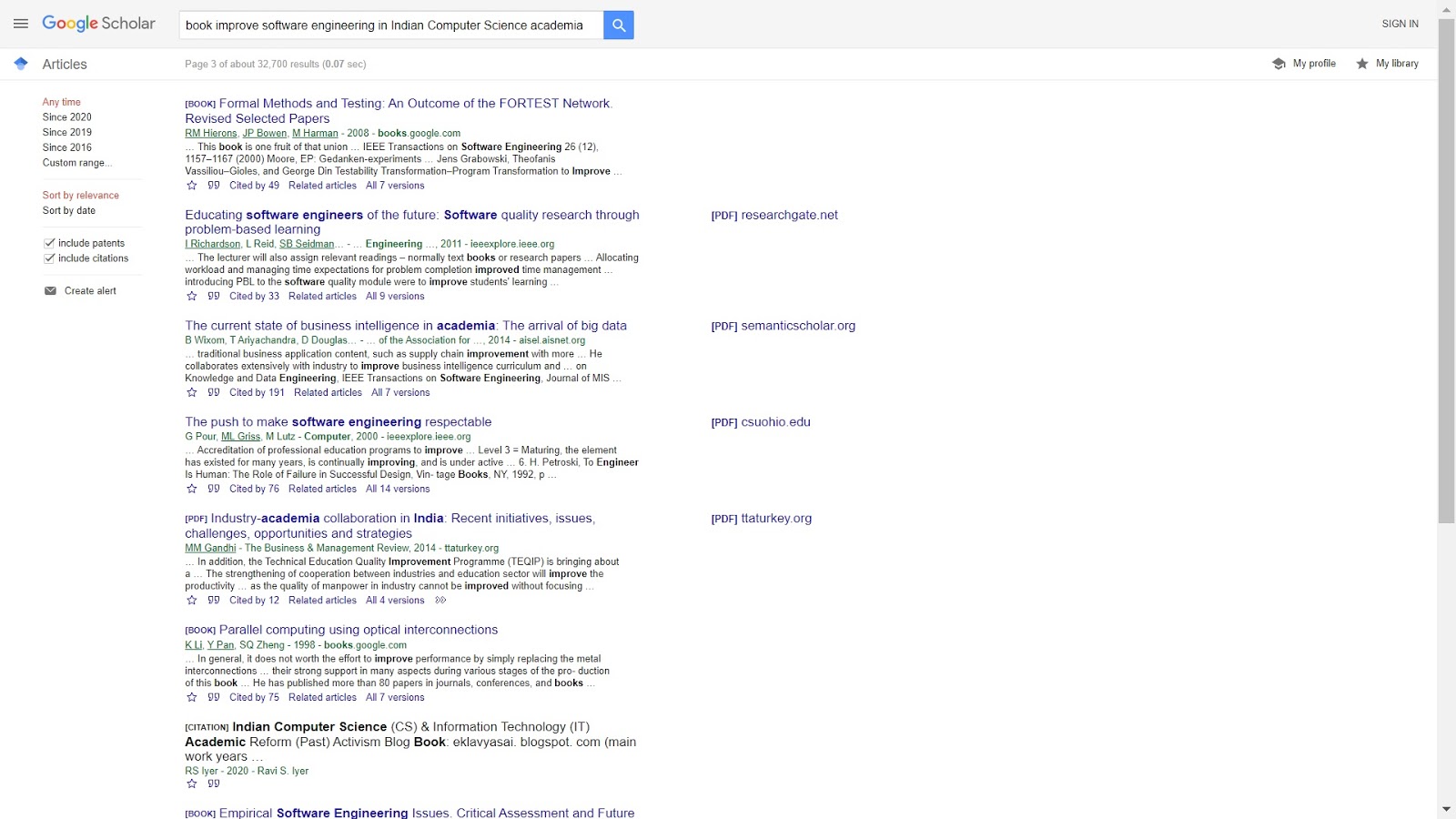The image is a screenshot of a Google Scholar search results page. At the top, the Google logo is displayed in its signature colors, followed by the word "Scholar." Nearby, three black menu bars are visible. Below, there's a prominent white search bar containing the query: "book improve software engineering in Indian computer science academia."

Beneath the search bar, on the left side, the word "Articles" appears. To the right, it shows the text: "Page 3 of about 32,700 results in 0.07 seconds." Further down, in purple, the text reads "Any time," and below in black, it lists time filters: "Since 2020," "Since 2019," "Since 2016." In green, there’s an option labeled "Custom range..." Additionally, in red again, it says "Sort by relevance," with an option underneath in black: "Sort by date." There are also checkbox options, both with blue check marks, labeled "Include patents" and "Include citations." A black envelope icon accompanies the "Create alert" option.

Following this, the screen lists search results:
1. **Book Form Methods and Testing and Outcome of the Fortis Network, Revise, Select Papers** - Authors in green, published in 2008, with "books.google.com" also in green. Description text in black.
2. **Educating Software Engineers of the Future: Software Quality Research Through Problem-Based Learning** - Authors in green, "researchgate.net" in purple, and description in black.
3. **The Current State of Business Intelligence and Academia: The Arrival of Big Data** - Authors and website "somaticscholar.org" in green, with description in black.
4. **The Push to Make Software Engineering Respectable** - Authors in green, description in black, with "csuo8ohio.ed" in purple.
5. **Industry-Academia Collaboration in India: Recent Initiatives, Issues, Challenges, Opportunities, and Strategies** - Authors and "ttaturkey.org" in green, description in black.
6. **Book: Parallel Computing Using Optical Interconnections** - Authors, book count, and website in green, description text in black.
7. **Indian Computer Science** - Title in black followed by CS and Information Technology in purple, "2020 Rabi S. Iyer" in green.

Near the bottom, partially cut off in purple, it reads: "Book: Imperial Software Engineering Issues, Critical Assessment and Future."